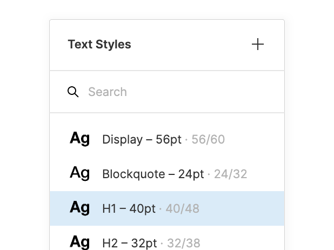This image shows a screenshot of a user interface panel dedicated to text styles. The top left corner of the panel is labeled "Text Styles" in black text. On the top right corner, there is a plus symbol icon. Below these elements, a small search bar displaying the word "Search" and a magnifying glass icon is visible.

The main section of the panel showcases four different font styles, each represented with the text "ag." These styles include:

1. "ag Display, 52pt"
2. "ag Block Quote, 24pt"
3. "ag H1, 40pt"
4. "ag H2, 32pt"

All instances of "ag" are depicted in bold lettering, with the "A" capitalized and the "g" in lowercase.